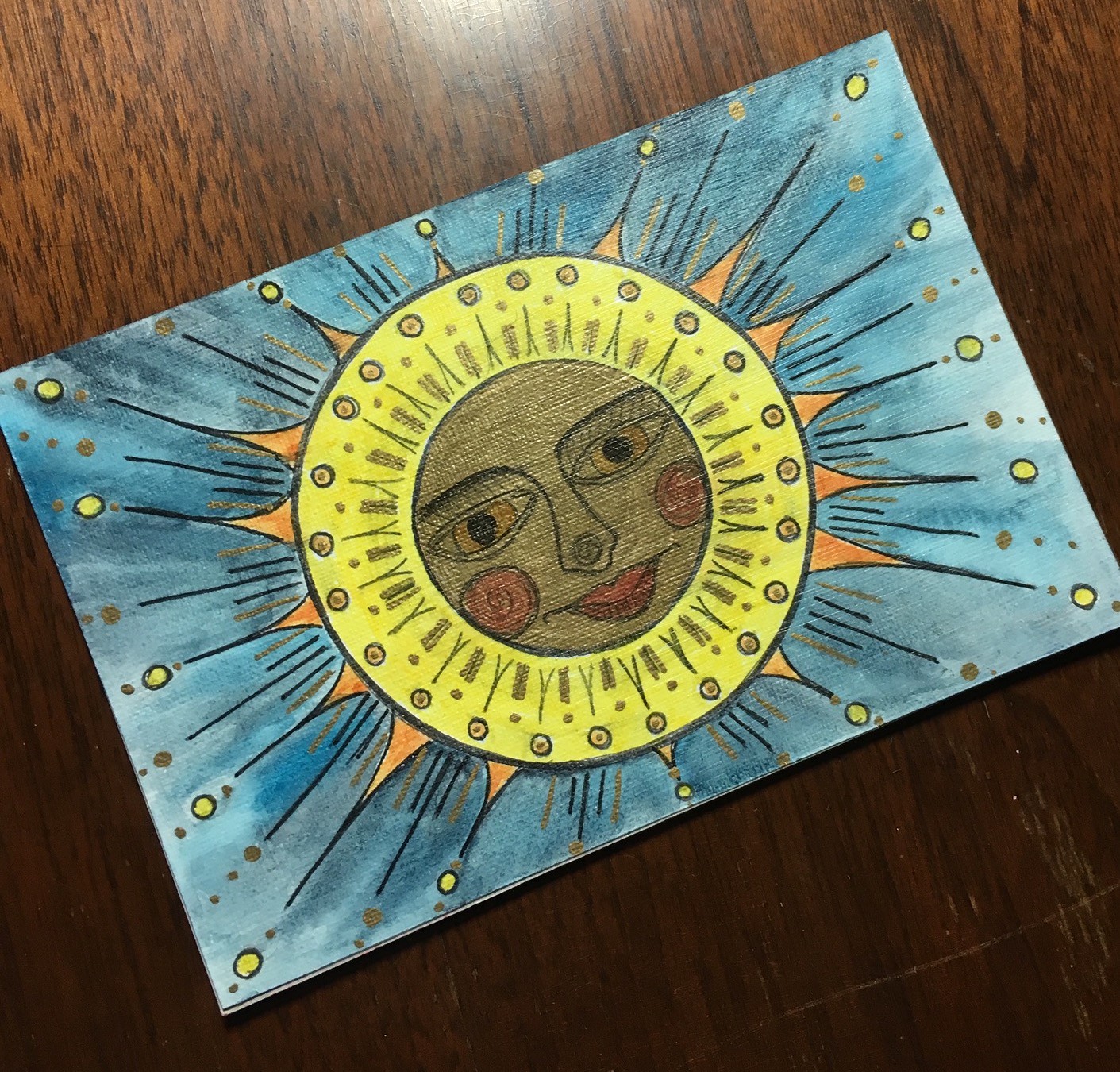This close-up color photograph captures a detailed drawing on a dark brown table with streaks of black and a light reflection at the top center. The artwork depicts a sun with an expressive face, featuring tan skin, prominent black eyebrows, golden eyes with black pupils, red circular blush marks on the cheeks, and red lips. The sun's central face is bordered by a large yellow ring adorned with small orange circles and brown and black lines. The sun’s rays, illustrated as alternating black lines and orange triangles, extend outward. The background showcases variegated shades of cyan and dark blue filled with numerous yellow circles and small brown dots, further enhancing the vivid, lively composition. The painting's canvas appears to extend beyond the photograph's frame, tilting from the bottom left to the top right corner.